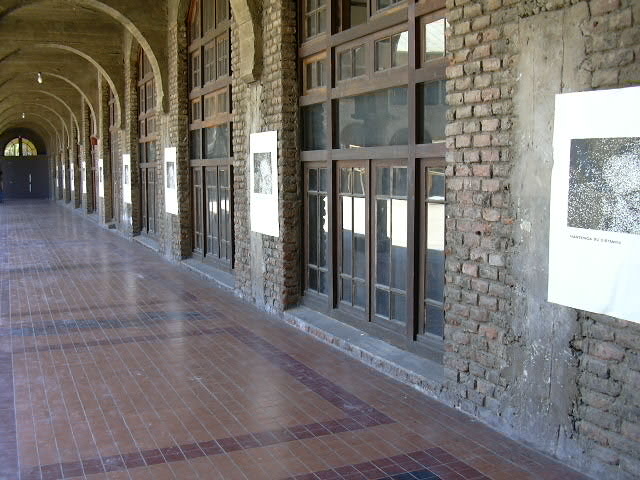This image, rectangular in shape, captures a photograph of an old, large brick building's exterior walkway or breezeway. The ceiling of the walkway is elegantly arched throughout its length. The floor is composed of small, shiny tiles, predominantly brown with red brick segments forming large square patterns as you proceed along the corridor. The walls show a mixture of red and brown bricks, and the space appears abandoned and dusty, void of any people.

On the right side of the walkway stands a series of large, floor-to-ceiling windows, each separated by brick columns adorned with large white posters. Each poster on these columns displays a black and white image with black text below, though the details are indistinguishable due to the distance. Suspended from some of the arched beams are light fixtures, festively illuminating the area. At the end of the walkway, a grand set of double doors with an arched top, including windows within the arch, marks the terminus of this inviting yet deserted corridor. Sunlight reflects through the windows on the left side, hinting at daylight and possibly indicating outdoor exposure.